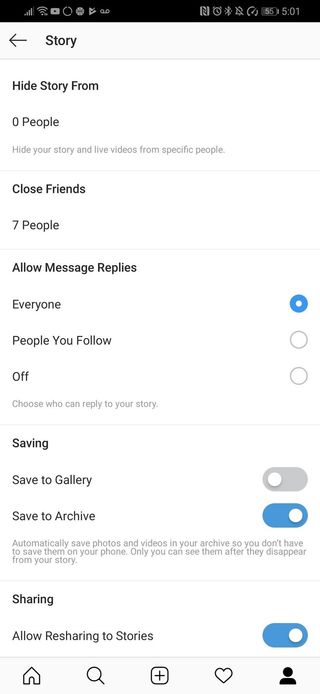A detailed screenshot from a cell phone displaying various settings options of a social media app interface. At the top, the notification bar shows icons for connection strength and battery life, indicating the time as 5:01. Below this, a gray strip with an arrow pointing left includes text that reads, "Hide story from," with an indication of zero people. It explains, "Hide your story and live videos from specific people."

A section labeled "Close Friends" shows that seven people are included, followed by "Allow Message Replies" with a highlighted blue circle marked "Everyone." Two additional options, "People You Follow" and "Off," are represented by blank circles. Small print clarifies, "Choose who can reply to your story."

The next section titled "Saving" features options for saving content. "Save to Gallery" is turned off, while "Save to Archive" is turned on, indicated by an oblong blue slider. An explanatory note mentions, "Automatically save photos and videos in your archive so you don't have to save them on your phone. Only you can see them after they disappear from your story."

Following this, the "Sharing" section shows "Allow resharing to stories," which is activated with a blue slider. Beneath these options, various icons are displayed, though not further detailed in the visible portion of the screen.